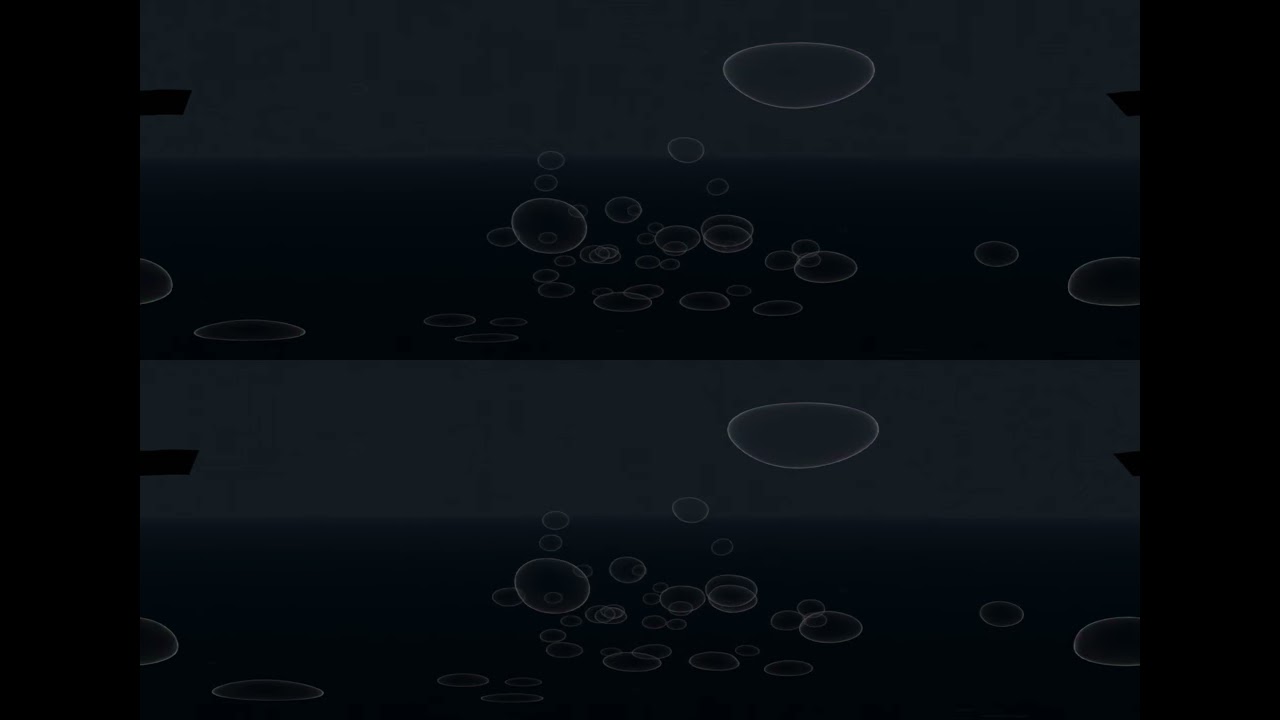The image features a graphical representation that primarily showcases a series of bubbles set against a water-like backdrop. There are two identical pictures positioned one above the other. Each picture is dominated by a group of bubbles with irregular, yet mostly circular shapes. The bubbles' boundaries are distinctly white. The background consists of two main color strips: a lighter blue strip at the top and a darker blue strip at the bottom. Most bubbles are concentrated towards the lower strip, with a few extending into the upper strip. Adding to the complexity, the image is bordered by vertical black strips on both the left and right sides. Despite an overall dark aesthetic, characterized by dark gray to dark blue hues, the bubbles appear vivid against the subdued color scheme. The bubbles seem to be centrally concentrated with a lighter dispersal towards the image’s edges, giving the impression of bubbles submerged within water.